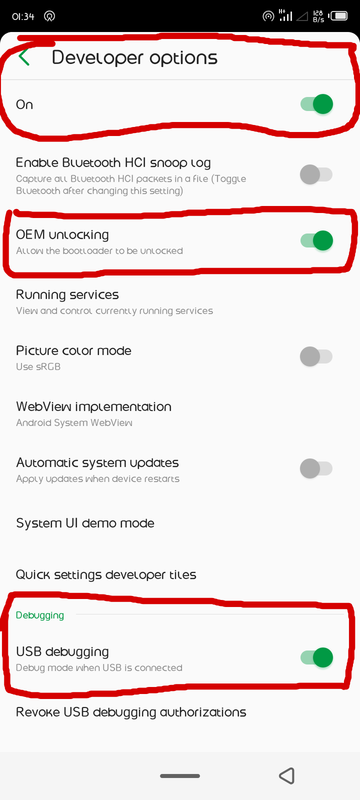This image is a detailed screenshot from a smartphone. The top features a black bezel displaying the time as 01:34 in a 24-hour format, accompanied by an icon resembling a person's silhouette within a circle. To the right of this is an unidentified target-like icon, a full signal strength indicator labeled "RX," and another empty signal strength icon, signifying dual-SIM functionality. Adjacent to these icons is text reading "128B-S," representing bits per second, and a battery icon showing approximately 70-80% charge.

In the foreground of the screenshot, a white menu is displayed, with a section circled in red ink. The first option, indicated by a left-pointing green arrow, reads "Developer Options." Below this, it shows "On" with a slider turned to the right, highlighted in light and dark green. The subsequent option, "Enable Bluetooth HCI Snoop Log," is turned off with a light gray slider. This item includes a description: "Capture all Bluetooth HCI packets and file (toggle Bluetooth after changing the setting)."

Another section, marked by a crudely drawn red rectangle, lists various settings. "OEM Unlocking" is on, with a green slider and a note underneath saying, "Allow the bootloader to be unlocked." Below this are options like "Running Services," "Picture Color Mode" set to use SRGB (with the slider off), "WebView Implementation" set to "Android System WebView," and "Automatic System Updates" also turned off.

In black text, it shows "System UI Demo Mode" and "Quick Settings Developer Tiles." Within another red rectangle, "Debugging" is highlighted in green. Below it, "USB Debugging" is bolded and followed by the description "Debug mode when USB is connected," with a green slider indicating it's on. Another option here is "Revoke USB Debugging Authorizations."

The bottom part of the screenshot is delineated by a light gray bezel, showcasing a black line and a black triangle pointing left.